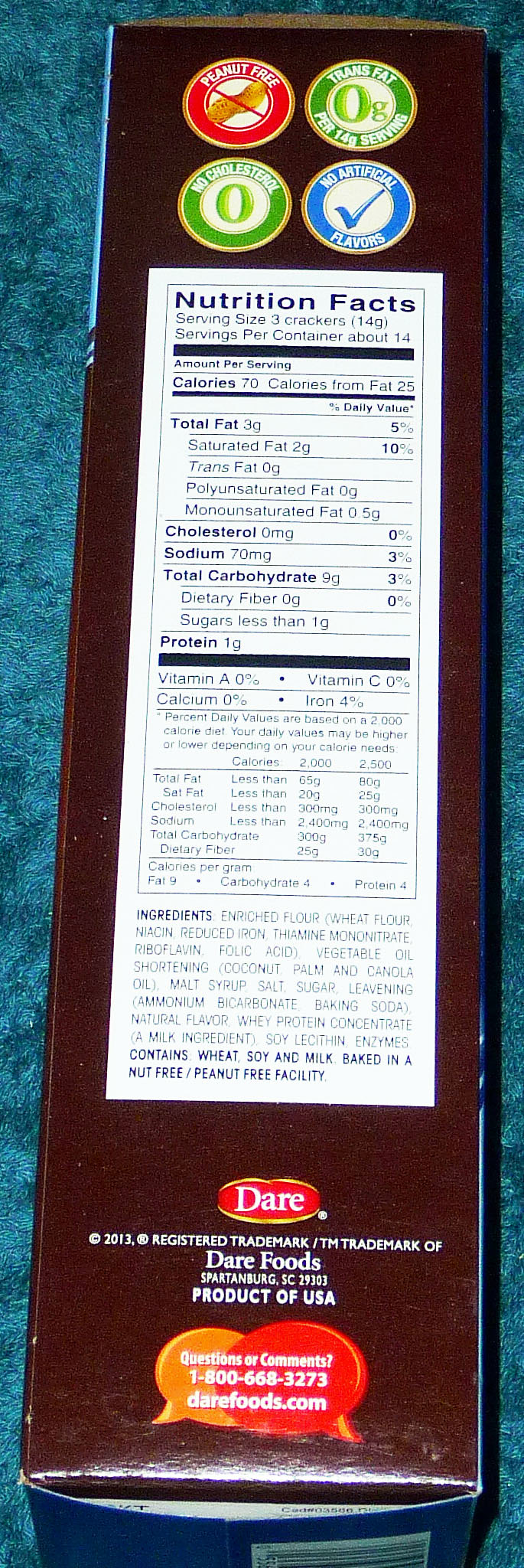This detailed photograph showcases the side of a box of crackers from the brand Dare, highlighted by distinct design elements and comprehensive nutritional information. The brand name "Dare" is prominently displayed, and there is a note indicating it is a 2013 registered trademark of Dare Foods, based in Spartanburg, South Carolina, with the additional accolade of "Product of the Year." At the bottom of the box, within a red bubble, the website "darefoods.com" is visible.

At the top of the box, there are several health-related icons and information circles. First, a red circle with a line through it and an image of a peanut signifies that the product is peanut-free. Below, a green circle indicates that there are zero grams of trans fat per 14-gram serving. Another green circle, located just beneath the peanut-free icon, declares the product has no cholesterol, symbolized by a zero in the center. Adjacent to this is a blue circle with a check mark, confirming that the crackers contain no artificial flavors.

Beneath these icons lies a detailed nutritional facts panel. It starts with the serving size, which is three crackers, and notes there are approximately 14 servings per container. The nutritional breakdown per serving includes: 70 calories, 3 grams of total fat, 0 milligrams of cholesterol, 70 milligrams of sodium, 9 grams of total carbohydrates, and 1 gram of protein. The list of ingredients follows this nutritional information.

The overall color scheme of the box consists of a brown background with a blue bottom, adding a distinctive visual appeal to the packaging.